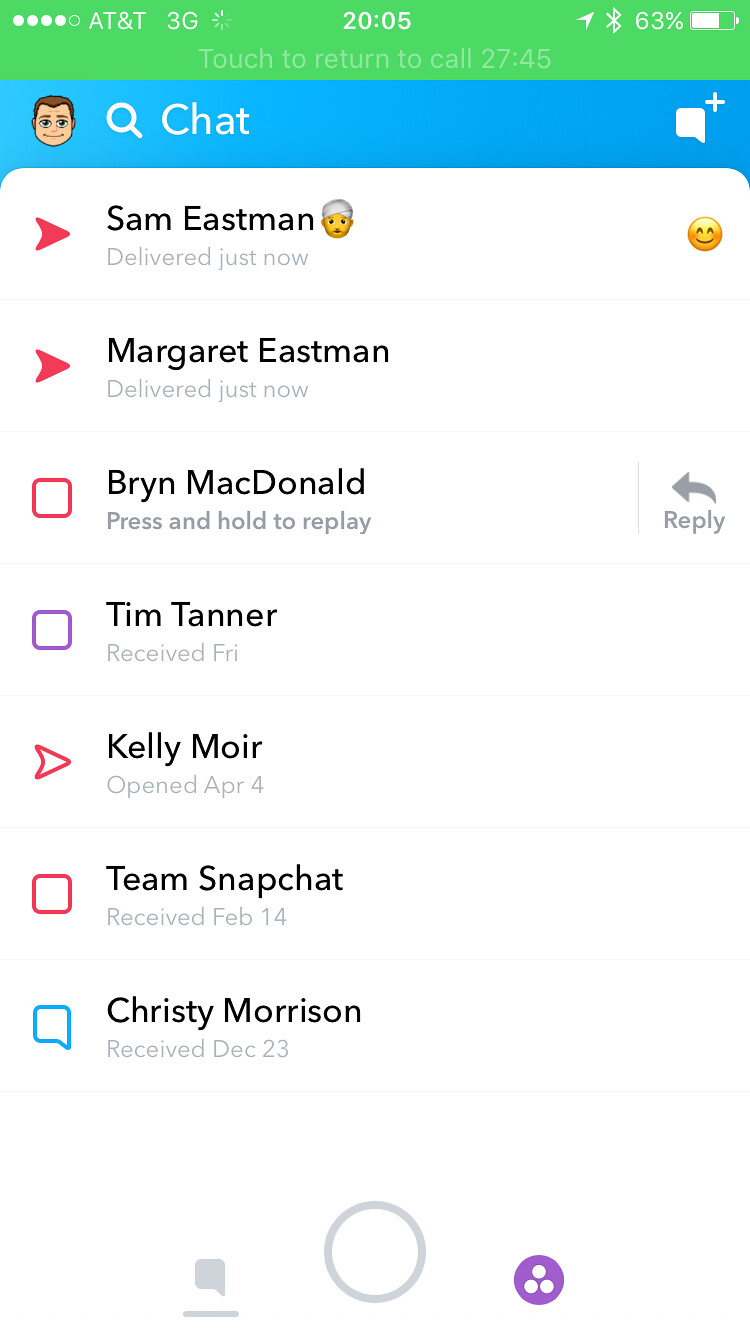This is a detailed color image screenshot from a Snapchat chat on a smartphone. At the top, the status bar displays AT&T 3G with a battery level at 63%. The time shows 20:05. An ongoing call notification reads, "Touch to return to call 27:45," indicating the call duration. Below the notification, the Snapchat interface shows names and message statuses: Sam Eastman and Margaret Eastman both have messages marked "delivered just now," Bryn McDonald shows "press and hold to replay," Tim Tanner's message was "received Friday," Kelly Moore's message was "opened April 4th," "Team Snapchat, received February 14th," and Christy Morrison's message was "received December 23rd."